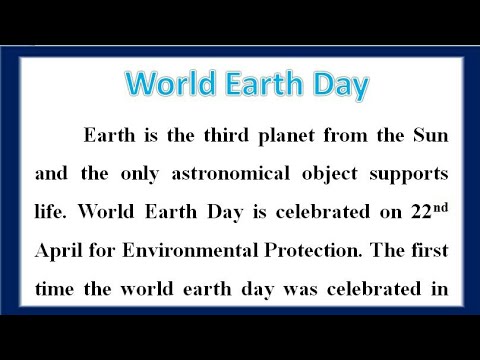A detailed description of the image reads: 

The image features the caption "World Earth Day" in light blue text prominently displayed at the top. The image is framed with a black border at both the top and bottom, with an additional dark blue border surrounding the main central area. The central section of the image features a clean design with a white background and predominantly black text. The text provides information about Earth and World Earth Day, stating: 

"Earth is the third planet from the sun and the only astronomical object known to support life. World Earth Day is celebrated on the 22nd of April for environmental protection." 

The caption appears to be cut off mid-sentence as it begins to explain the history of World Earth Day, ending abruptly with: "The first time the World Earth Day was celebrated in..." 

Despite the incomplete nature of the text, the image effectively communicates key details about the significance of Earth and the annual celebration dedicated to its protection.